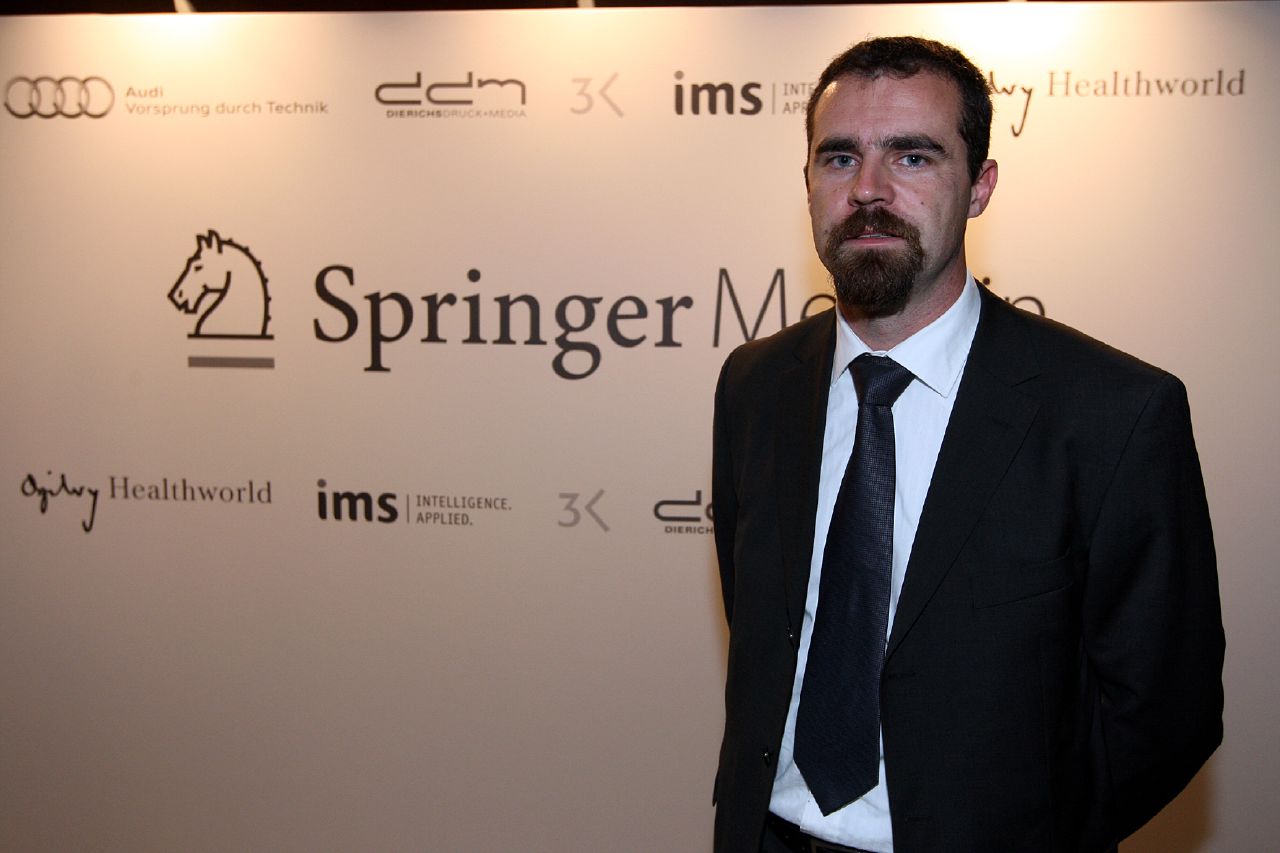A man stands slightly off-center to the right of a white backdrop in this image. He is facing the camera with his arms behind his back, showcasing his black suit jacket, which is unbuttoned, revealing a white button-down shirt and a dark tie. The man has short brown hair, a brown goatee, and blue eyes. The backdrop behind him features various logos and company names in black and grey. Prominently to the left of him, the word "Springer" stands large, accompanied by a horse head logo resembling a chess piece in a side profile view. In the upper left corner, the Audi logo with the text "Vorsprung durch Technik" is visible. Above his right shoulder, the words "Health World" can be seen, and further down, additional logos and texts such as "Intelligence Applied" and "IMS" are spread out. The setting seems to depict a promotional or formal event, possibly a red carpet, with spotlights illuminating the banner.